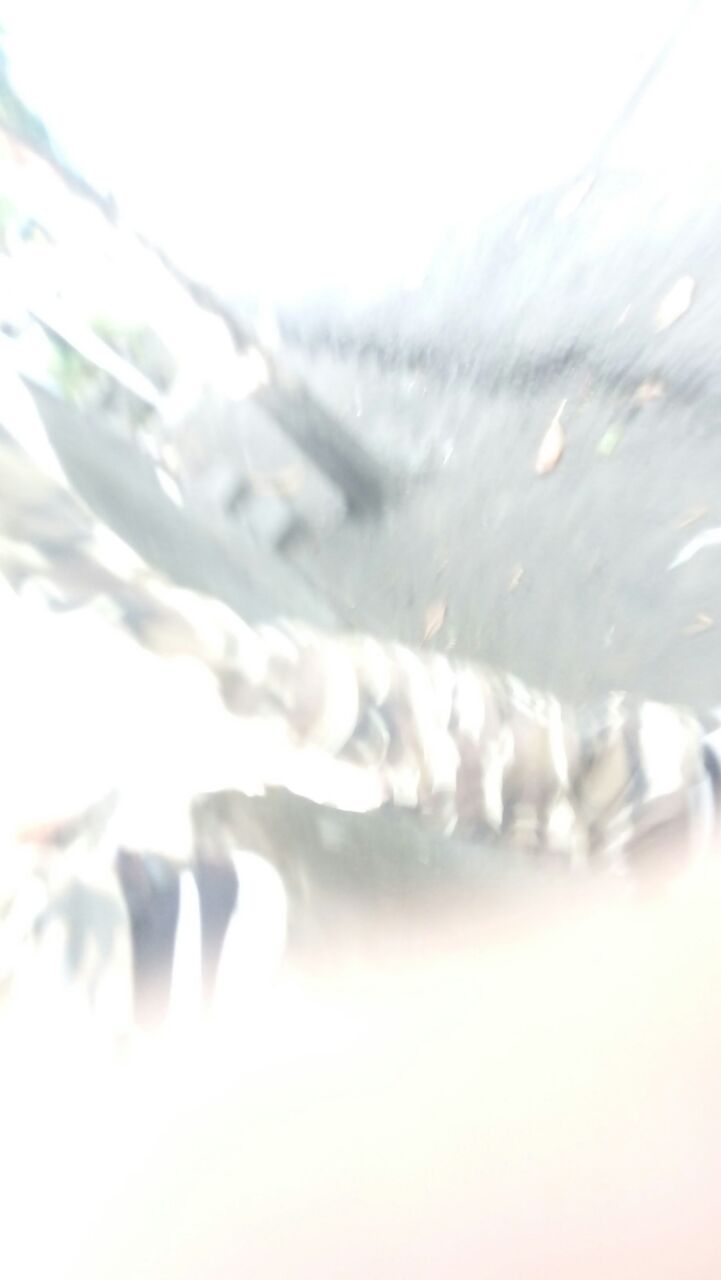This image is predominantly vertical, with a glaring overexposure rendering the scene almost completely indistinguishable. The image radiates a blinding whiteness, akin to the reflective brilliance of snow under intense light. The bottom right-hand corner is a solid, glaring white, which merges into an amorphous blur on the left side, suggesting the possibility of an outdoor scene blanketed in snow or suffused in bright sunlight. Intruding into the white void from the left, there is an obscure shape that could be interpreted as either a leg or a towering structure, paired with a potential walkway beneath. The overwhelming bright light and ambiguous forms make it challenging to ascertain the exact setting. Hints of orange at the bottom edge provide a slight contrast to the pervasive whiteness. The overall impression is one of an outdoor scene, possibly in winter, engulfed in dazzling brightness and obscured by overexposure.